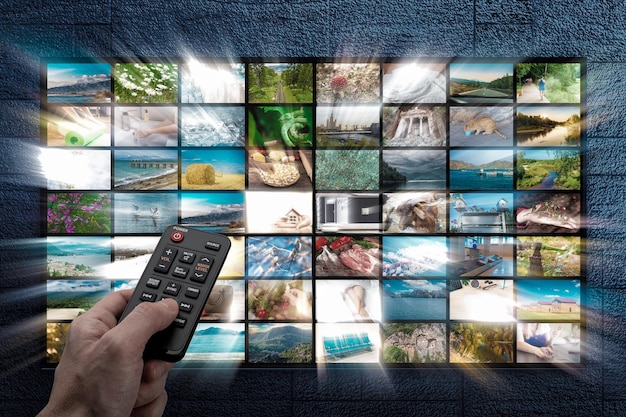This image presents a detailed collage of various TV channels, each showcasing unique content. Spread across a wall that is seven screens high and eight screens wide, no two channels display the same imagery. The top left screen features a majestic mountain, while two rows down on the right, an image of an animal can be seen. These screens display diverse visuals ranging from scenic outdoor landscapes, such as beaches and parks, to ancient architectural wonders like Petra, as well as colorful flowers and other vibrant scenes from around the world. 

At the bottom left corner, a hand holding a black TV remote is prominently featured. The remote is detailed with several buttons, including a distinct red on/off button, symbolizing the act of browsing through these intriguing channels. The composition of the image gives a glowing, almost shining effect, emphasizing the engaging and varied programs available for selection. The overall graphic conveys a dynamic viewing experience, inviting viewers to explore and choose from the multitude of captivating channels offered.